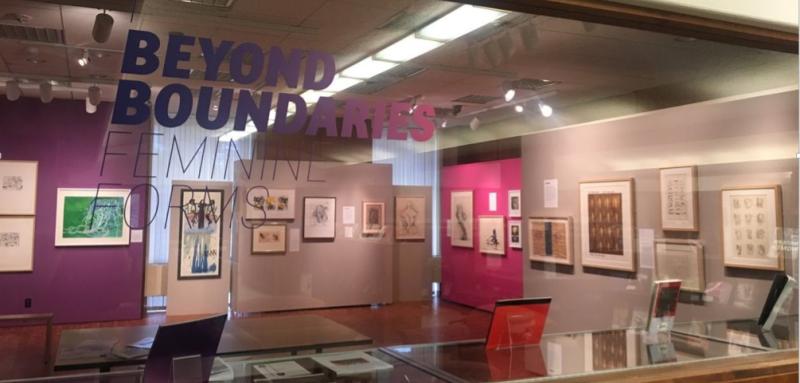The image captures a view from the outside, looking through a large glass pane into a brightly lit gallery or shop. On the glass, bold sans-serif text reads "Beyond Boundaries" in a striking purple to pink gradient, with "Feminine Forms" written below in a much thinner font. Inside the space, polished wooden floors lead the eye to a variety of colorfully painted pop-up walls—light pink beige, bright pink, and dark purple—each displaying more than 20 framed artworks. These artworks are meticulously organized, some accompanied by descriptive text. The ceiling is lined with typical classroom or office lighting, augmented by hanging lights that spotlight individual pieces. Directly behind the glass, near the front, is a long glass-topped counter adorned with unidentifiable items that resemble photo holders or electronic devices.